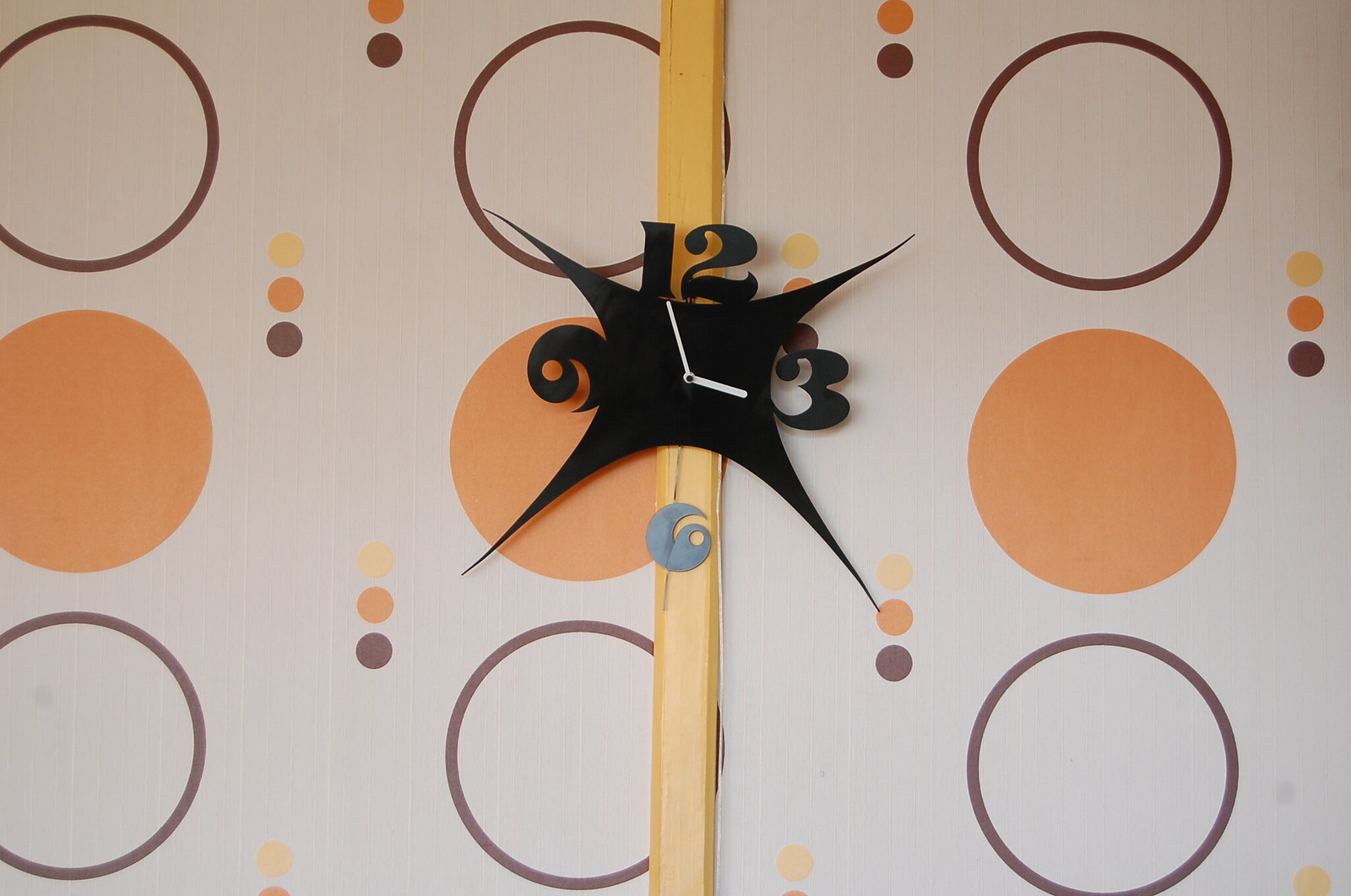The image showcases a uniquely designed clock face, characterized by its minimalist aesthetic and bold stylistic elements. The clock features only the numbers 12, 3, 6, and 9, presented in highly stylized Arabic numerals. These numbers, along with the black background of the clock face, form an intricate pattern reminiscent of three interconnected parabolas, creating a shape similar to an X with a thick center. This visual arrangement leads to a symmetry that leaves gaps between the numbered points, enhancing the focus on the design.

The hour and minute hands of the clock are both white and have rounded corners, providing a clean contrast against the black face. The clock is mounted on a piece of wood, which is in turn attached to a wall adorned with distinctive wallpaper. The wallpaper features a repeating pattern of larger circles in shades of brown and orange, interspersed with columns of smaller circles. These smaller circles appear in sets of three, alternating between tan, orange, and dark brown. The overall color scheme and pattern of the wallpaper add a retro yet warm atmosphere to the setting.